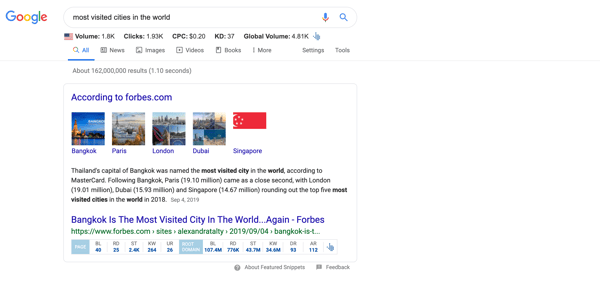The image depicts a Google search results page. In the top-left corner, the Google logo is prominently displayed. To its right is the familiar search bar with the query "most visited cities in the world" typed inside. Adjacent to the text within the search bar are a microphone icon and a magnifying glass icon representing voice search and standard search functions respectively.

Below the search bar, metrics such as volume, clicks, CPC (Cost Per Click), KD (Keyword Difficulty), and global volume are listed. Directly beneath these metrics is a horizontal menu featuring options from left to right: "All" (which is currently highlighted), "News," "Images," "Videos," "Books," "More," "Settings," and "Tools."

Further down, in small grey text, the page indicates there are "162 million results." Immediately below this text, a blue hyperlink states "according to Forbes.com," listing Bangkok, Paris, London, Dubai, and Singapore as the top five most visited cities. Above each city name, there is a corresponding square image. Additional information in small black text follows, mentioning the date "September 4th, 2019."

The next section begins with a search result headline "Bangkok is the most visited city in the world, again - Forbes." Underneath this headline is a green website link. Additional information and categories are listed below this link with numbers in blue and their descriptive labels in light grey.